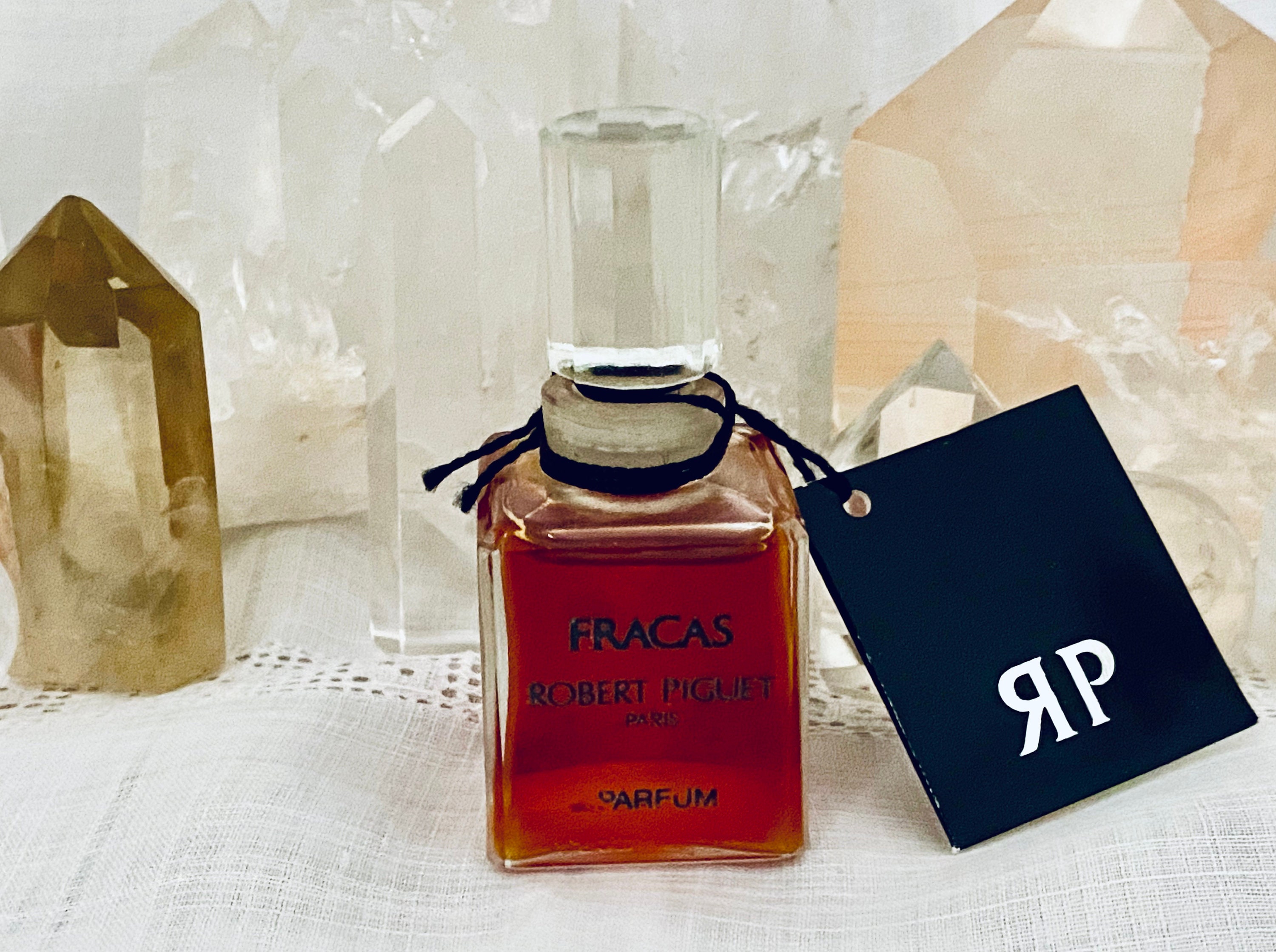This photograph features a vintage square glass bottle of Robert Piguet's Fracas perfume, centrally positioned. The bottle contains a dark honey or amber-colored liquid and is topped with a tall, cylindrical lid. A distinctive black or navy blue tag, bearing the reversed 'R' next to a properly facing 'P', is affixed to the right-hand side of the bottle. Surrounding the perfume are several upright quartz crystals: a dark golden one, resembling citrine or smoky quartz, to the left, and a pink-tinted quartz to the right in the background, with additional clear crystals. The image, slightly out of focus and grainy, evokes a nostalgic 1980s aesthetic. The scene is set upon a cloth, possibly a lace-trimmed tablecloth, creating an elegant display that hints at a vintage advertisement or sales listing.